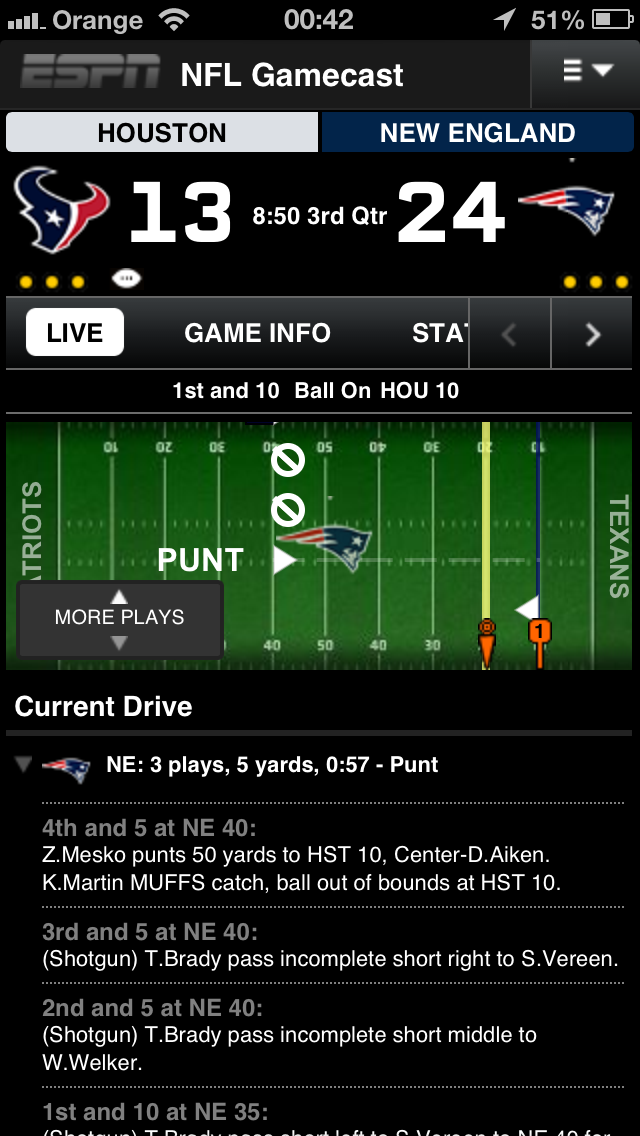The image appears to be a screenshot from a smartphone app, specifically displaying an ESPN NFL GameCast interface. At the top of the screen, common smartphone status icons are visible, including a white signal bar, a label reading "orange" between signal bars for Wi-Fi and cell service, the time displayed as 00:42 in the center, and a battery icon at 51% on the right. Below this, the ESPN logo is showcased with "NFL GameCast" in white text against a dark gray background. 

The game details feature the teams Houston (left, white background) and New England (right, dark blue background) with their respective logos—Houston's bull head silhouette in blue, white, and red with a star for an eye, and New England's 2D Patriot head in red, white, and blue. The scores are prominently displayed: Houston 13, New England 24, with the game time indicating 8:50 in the third quarter. Additional in-game options like "live," "game info," and partially visible "stats" are listed below.

The display also provides a detailed breakdown of the game's progress. It mentions "First and 10, ball on HOU 10," and features a 2D football field image. The field is marked from the 10-yard line to the 50-yard line, and back to the 10-yard line of the opposing team, with a Patriots logo at midfield, indicating New England's home field. A yellow marker shows the ball on Houston’s 10-yard line, and the first down marker at the 20-yard line.

At the bottom of the screen, the current drive section lists New England’s recent plays (three plays for five yards in 57 seconds ending in a punt) along with other drive statistics, presented in white text on a black background. Some of the game drives are partially cropped out at the bottom, adding context to the live football game viewing experience offered by the app.